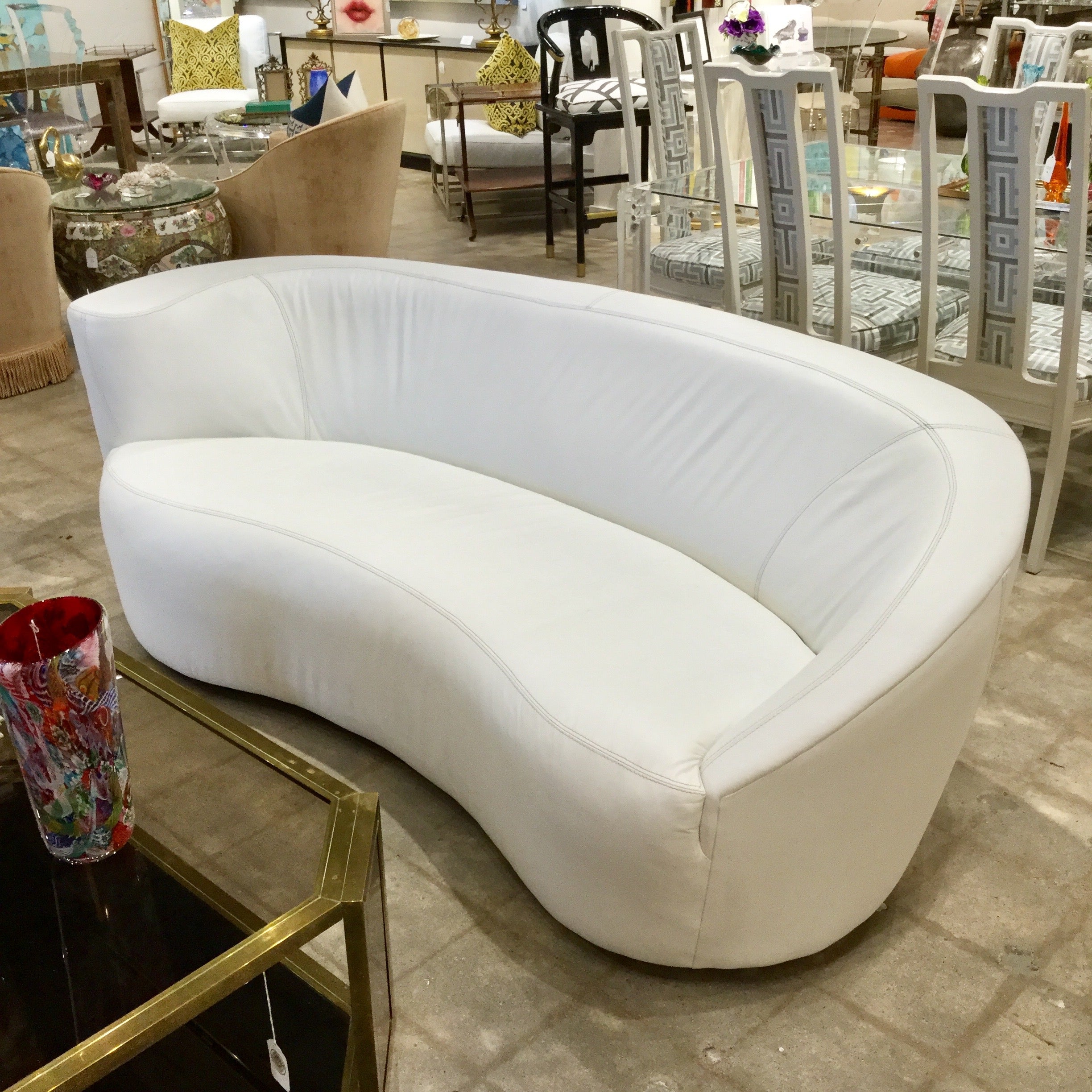This image depicts an interior setting, likely a furniture store, showcasing an array of furnishings on a brown, brick-shaped tile floor. Central to the image is a white, curvy sofa with clean lines and a semi-circular design. Beside this sofa, there is a glass-top coffee table with a gold trim. Surrounding the sofa, various pieces of furniture are visible, including brown and white chairs, among them a distinctive white chair with a gold pillow positioned in the corner.

Behind the sofa stands an elegant dining table with tall, cream-colored chairs featuring gray designs, also capped by a glass tabletop. Additionally, there is a brown table and several round wooden chairs dispersed throughout the scene. Within the space, a unique piece of furniture—a cabinet—displays a picture frame with an image of a pair of lips. The room is filled with numerous other items that suggest this could be a showroom or a retail environment, characterized by plentiful furniture tags indicative of sale items.